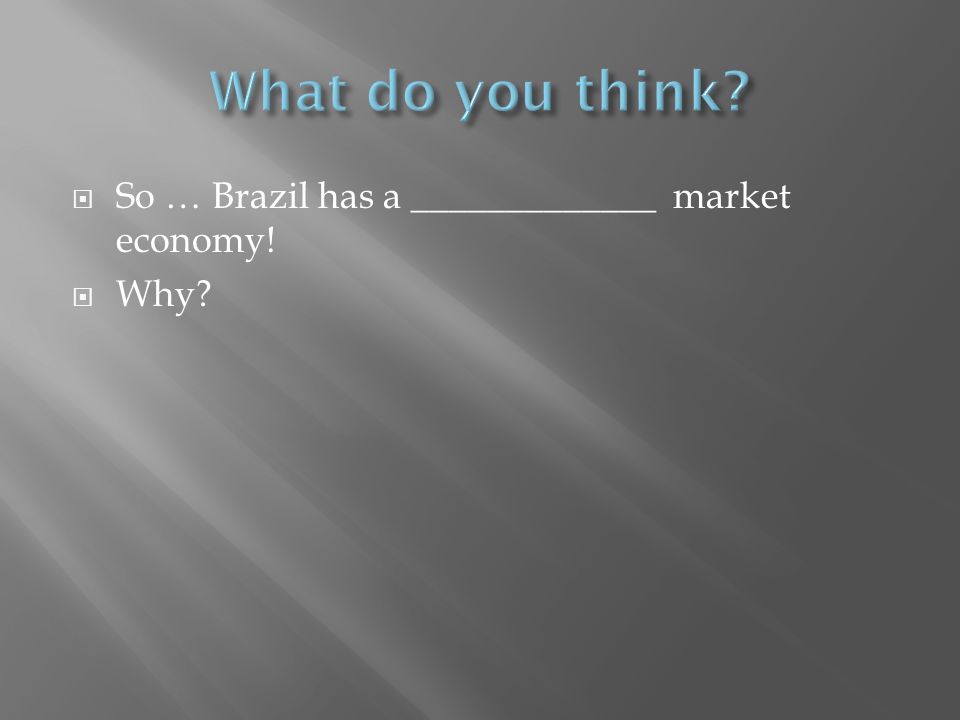The image depicts a PowerPoint slide with a predominantly gray background, illuminated by a light source coming from the left. At the top of the slide, there is a prominent question written in thin, light blue font that reads, "What do you think?" Below this, in the same light blue font but smaller, is a prompt: "Brazil has a ____ market economy."

Additionally, there is another prompt below the fill-in-the-blank sentence. This section features two bullet points, each enclosed in a white square. The first bullet point reads: "So..." with an ellipsis, and the second bullet point simply states: "Why?" Both bullet points are in white font, maintaining a thin and unbolded style consistent with the rest of the text on the slide.

This PowerPoint slide is clearly designed to provoke thought and discussion by asking the audience to identify the type of market economy Brazil has and to provide reasoning for their answer.